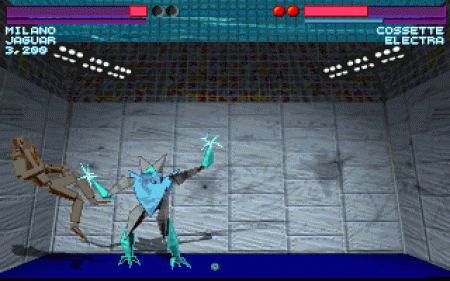This screenshot captures an intense moment in a video game set in a square fighting arena. On the left, a tan-colored robot is depicted mid-air, seemingly propelled backward from an impact. At the center of the scene stands a formidable opponent, a hybrid of monster and robot. This towering figure has three distinctive shark-like toes and legs that transition from gray at the top to blue at the bottom. Its forearms are also blue, ending in what appear to be sparklers. The creature's chest features a prominent blue, upside-down triangle, and it has two horn-like projections on its head, contributing to its menacing appearance. The dynamic action and detailed character designs make this screenshot a vivid representation of the game's thrilling battles.